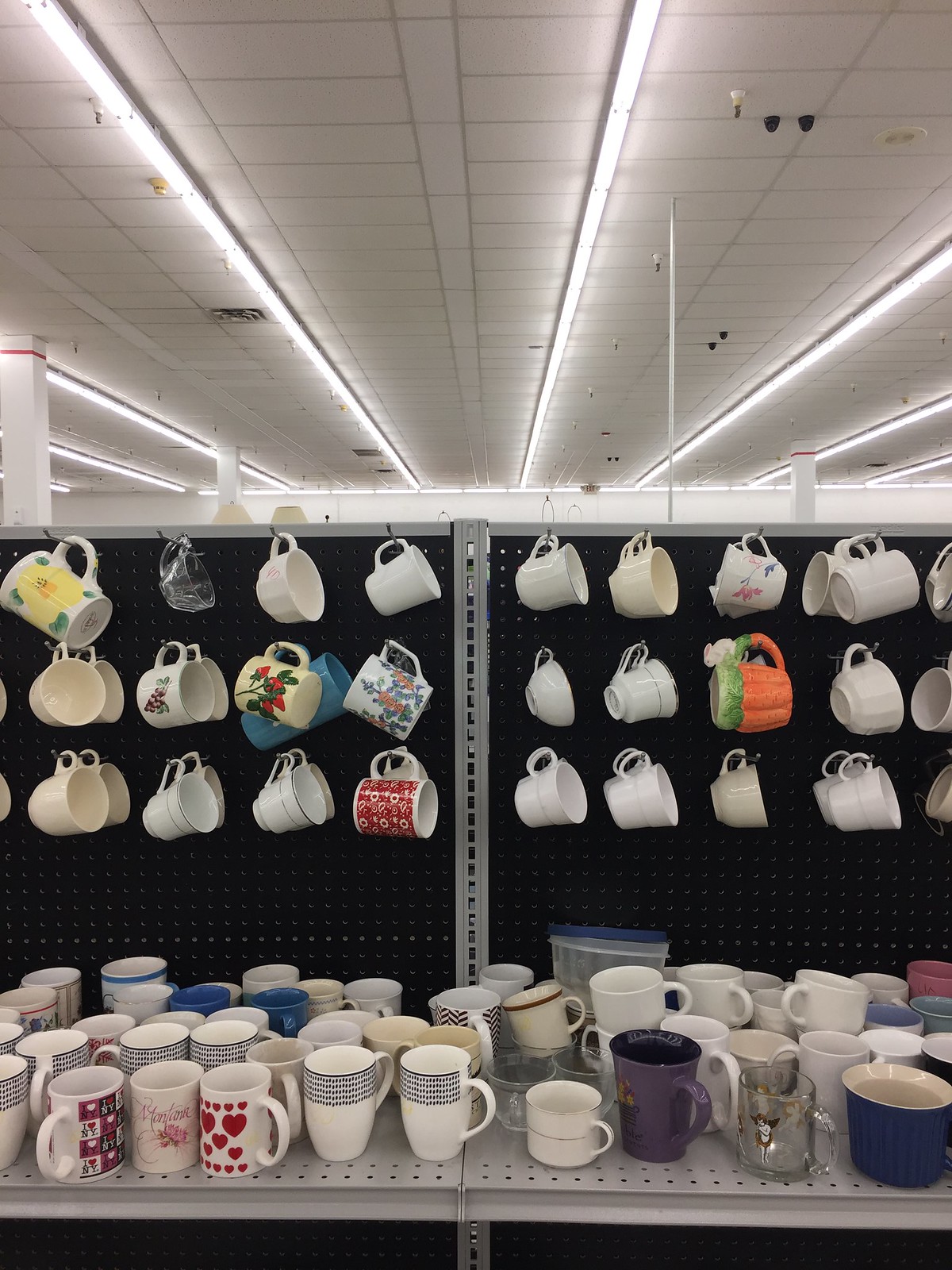The image depicts the interior of a thrift store, highlighting a section dedicated to coffee mugs. The ceiling is lined with long rows of fluorescent lights embedded in ceiling tiles, casting a bright, even illumination over the area. The focal point is a pegboard shelving system running along the lower half of the image. The pegboard accommodates a neat arrangement of three horizontal rows and eight vertical columns of hooks, each hook exhibiting a distinctive coffee mug. The mugs vary in size and style, with many being plain white, while others are more unique, such as a pumpkin-shaped mug. Below the pegboard, a gray metal shelf holds an eclectic assortment of additional mugs. This lower shelf features a range of designs, including white mugs with blue dotted borders, a mug adorned with multiple hearts, and another with a pink and purple picture. There are also solid-colored mugs, such as a striking purple one and a large blue one, adding a splash of color to the display. The overall scene captures the diverse collection available for shoppers, emphasizing the variety and charm typical of a thrift store.